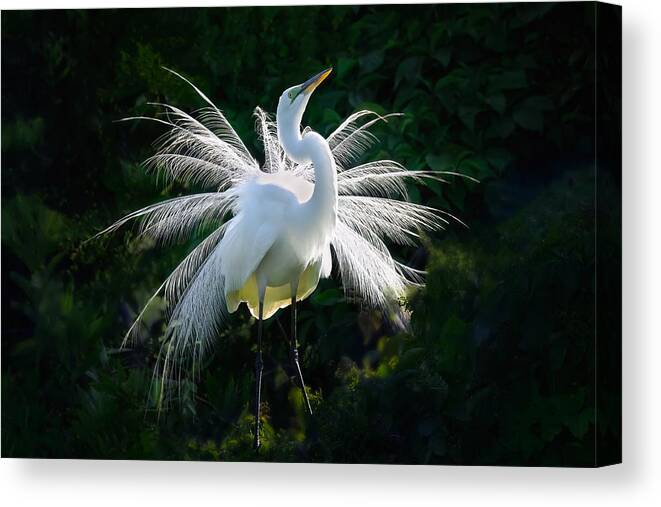This image features a beautifully captured moment of a tall, elegant bird standing amidst lush foliage. The bird, predominantly white with a tall stature, has black legs and an orange-tinted beak. It stands on a dark green to almost black background filled with leaves, suggesting a natural, possibly forested setting. The bird, resembling a swan or a similar species, is actively extending its neck upwards towards the sky, exuding grace. Its tail feathers are reminiscent of a peacock's fan, white and wispy, gracefully splayed out behind it with a dynamic, almost swirling motion. This print, displayed on a canvas with a white background, seems poised for sale on a website, offering a horizontal image with a captivating and serene composition.